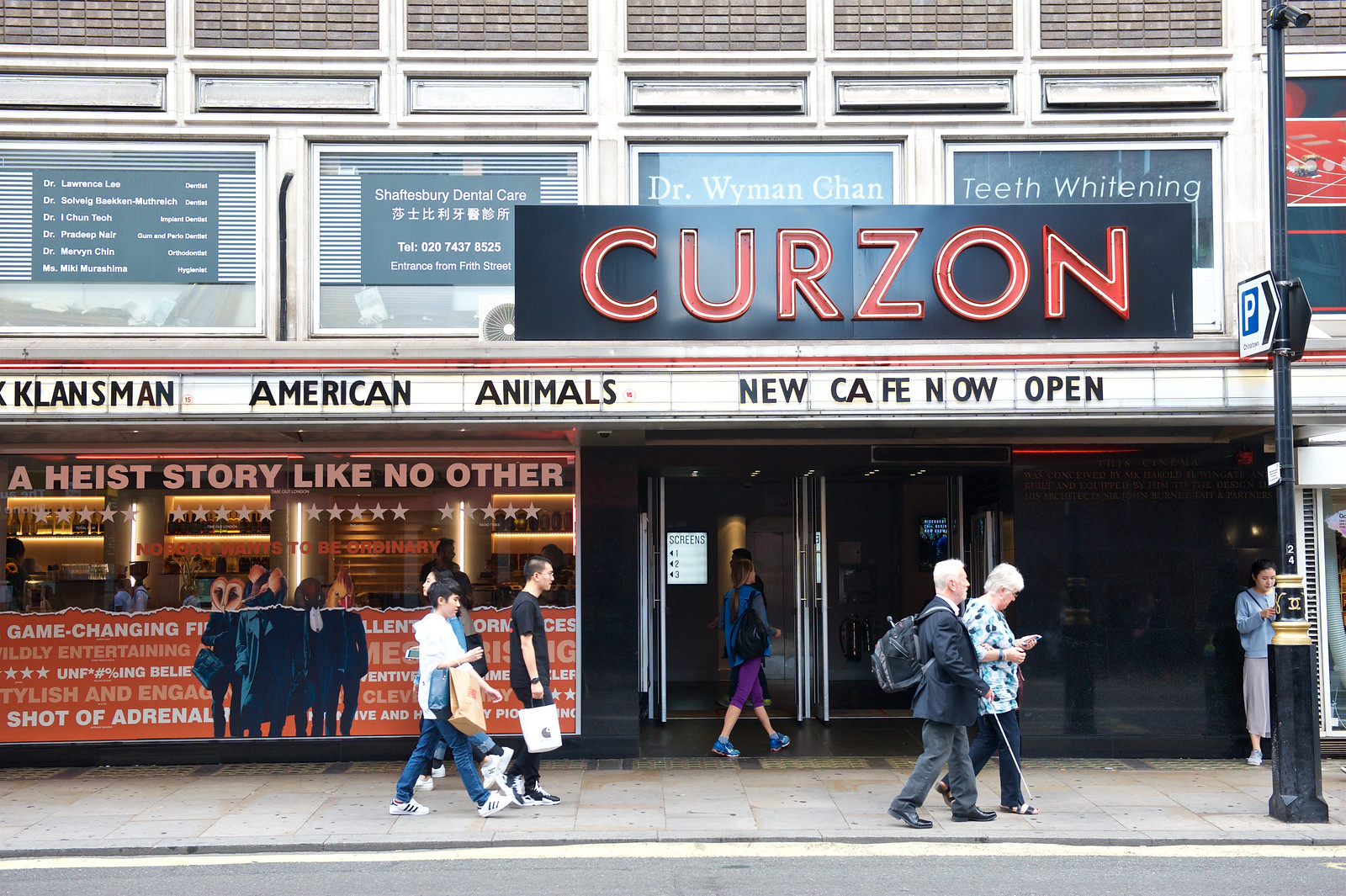The image depicts the storefront view of an establishment with a suggestion of it being a cinema or a newly opened café. At the top of the storefront, the name "CURZON" is displayed prominently in large, bold red letters. Below this, there is a sign reading "Klansman," "American Animals," and "New Cafe Now Open," suggesting both movie titles and a possible café opening. The storefront features large glass windows on both sides and centrally located double-paned glass doors. Above the doors, there is additional signage in black text with statements including "Dr. Win Min Chan," "Teeth Whitening" on the right, and "Shaftesbury Dental Care" on the left. People are seen walking in front of the store, including a girl appearing to enter and an elderly couple, the man using a cane. The setting includes a street with visible sidewalk and a small portion of the road. The entire scene suggests a bustling area with commercial activity and pedestrian traffic.